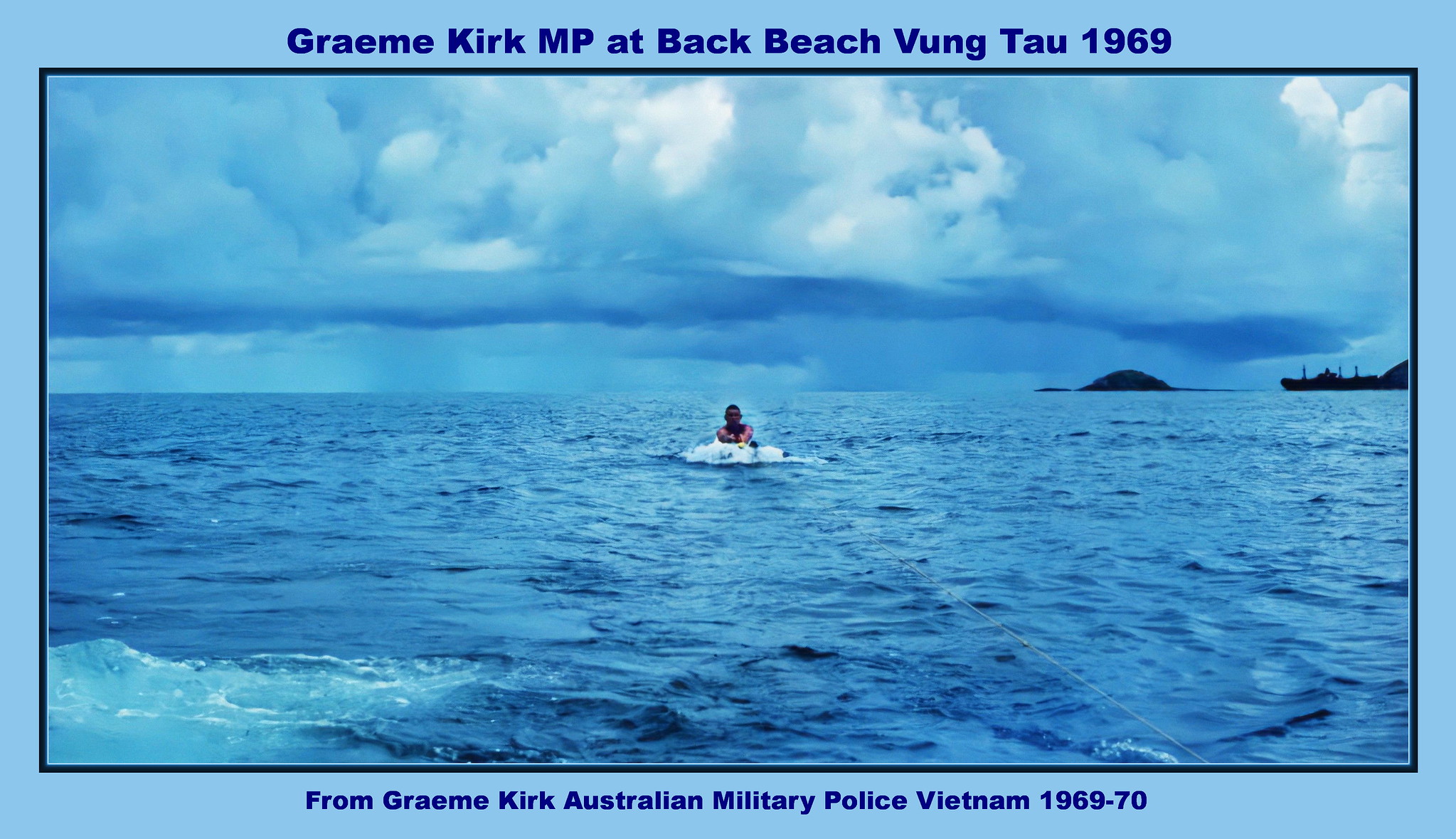The photograph, framed by a light blue outer border and a thin black inner border, captures a scene at Back Beach, Vung Tau, in 1969. In the vibrant turquoise waters, an individual, identified as Graeme Kirk MP, is seen on a white flotation device being towed by a boat barely visible at the end of a thin white string. The ocean, though dark blue and somewhat rough with noticeable waves, contrasts beautifully against the overcast sky filled with numerous clouds. In the background, a silhouetted mountainous area adds depth to the scene. The top of the picture features blue text stating “Graeme Kirk MP at Back Beach Vung Tau 1969," while the bottom reads, “From Graeme Kirk, Australian Military Police, Vietnam 1969-70.”